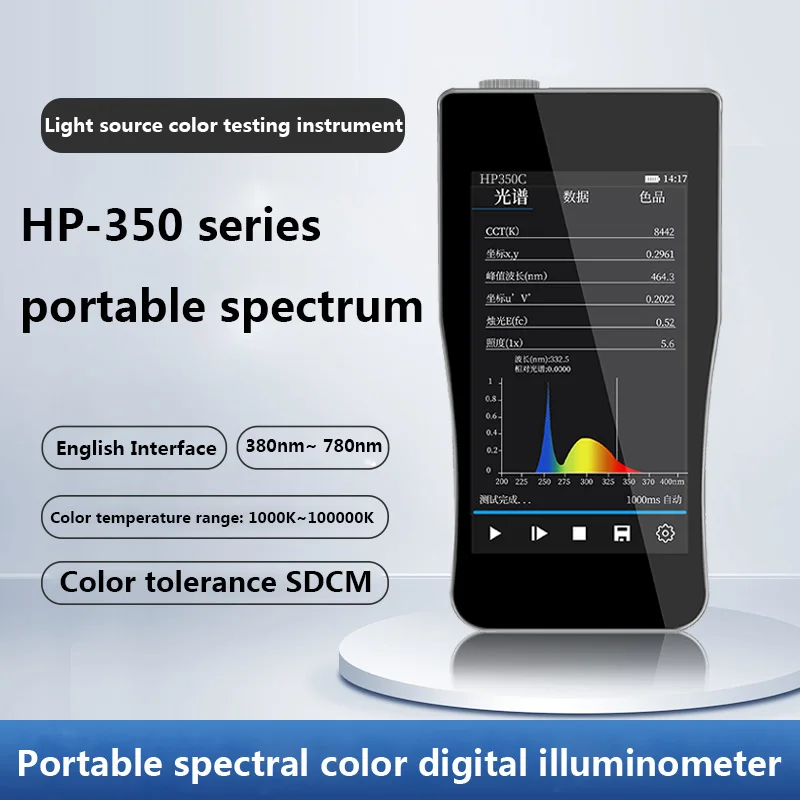The image is an advertisement featuring the HP 350 Series Portable Spectrum, a sophisticated light source color testing instrument. This handheld device resembles a slender cell phone with a bright screen displaying a detailed spectral graph ranging from blue to red, covering the entire color spectrum from 380 nanometers (nm) to 780 nm. The device features color peaks and valleys from ultraviolet to infrared wavelengths. The screen interface, primarily in English but with some Oriental characters, provides real-time data such as battery power, time (notably 14:17), and the label "HP 350C" at the top left. Additionally, the graph includes a play button, possibly for video animation or further analysis.

The ergonomic design is accented by a gray background and a prominent blue band at the bottom with white lettering that reads "Portable Spectral Color Digital Illuminator." Below the device's name, the advertisement lists its technical specifications: a color temperature range from 1000K to an impressive 100,000K and a color tolerance of SDCM. This makes it an essential tool for professionals evaluating various light forms and sources.